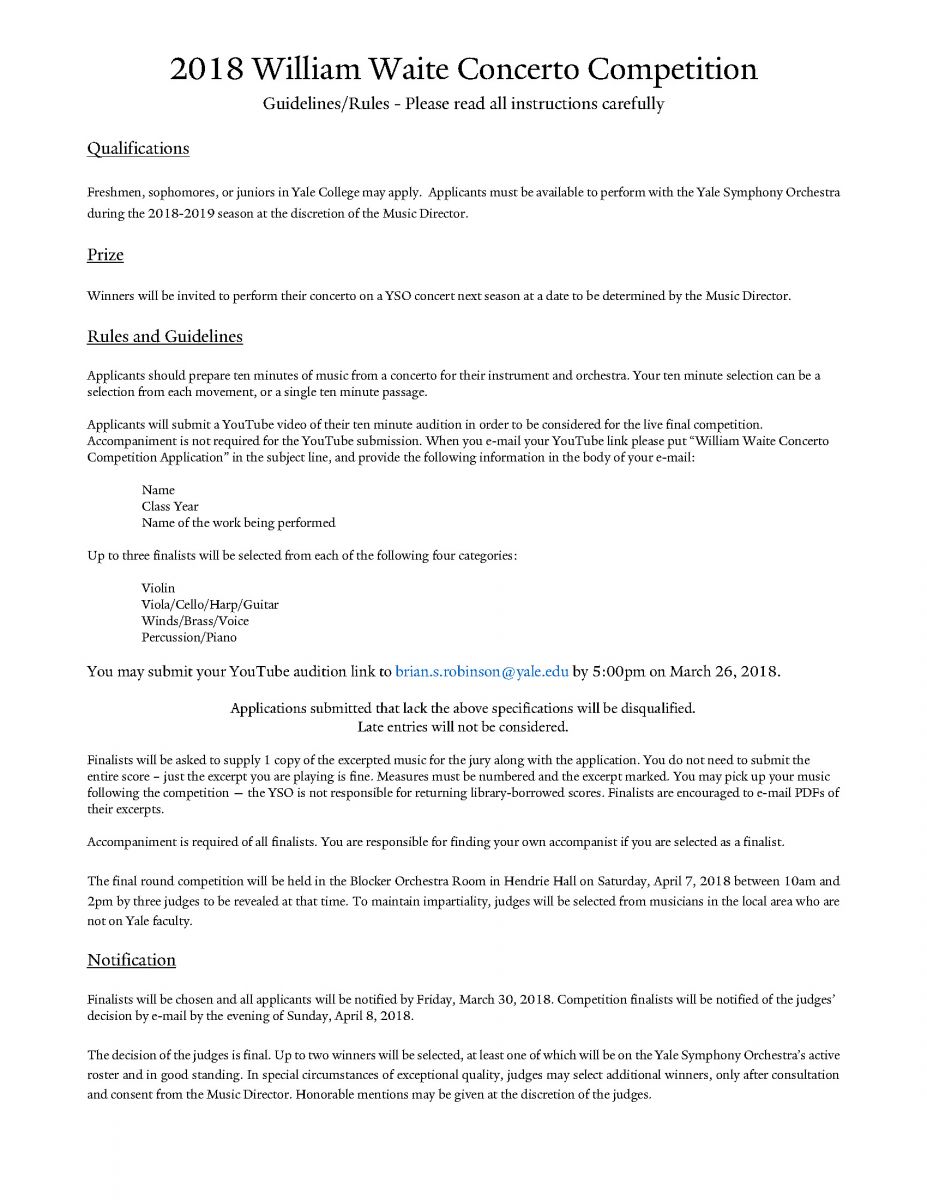This image is a detailed announcement for the 2018 William Waite Concerto Competition at Yale College. The text outlines the competition's guidelines and rules, emphasizing the importance of reading all instructions thoroughly. The qualifications specify that only freshmen, sophomores, or juniors at Yale College are eligible to apply, and applicants must be available to perform with the Yale Symphony Orchestra during the 2018-2019 season, with participation contingent upon the music director's discretion.

The prize for the competition is the opportunity for winners to perform their concerto with the Yale Symphony Orchestra in the next season, with the performance date determined by the music director. Applicants are required to prepare and present 10 minutes of music from a concerto appropriate for their instrument and orchestra. This 10-minute submission can either be a complete movement from the concerto or a selection from different movements, compiled to meet the time requirement.

Further details include the necessity for applicants to provide their name, class year, and the name of the work they will perform. Up to three finalists will be selected in each of the following categories: violin, viola, cello, harp, guitar, winds, brass and voice, percussion, and piano.

The submission process involves sending a YouTube audition link to Brian S. Robinson at brian.s.robinson@yale.edu by 5 p.m. on March 26, 2018.